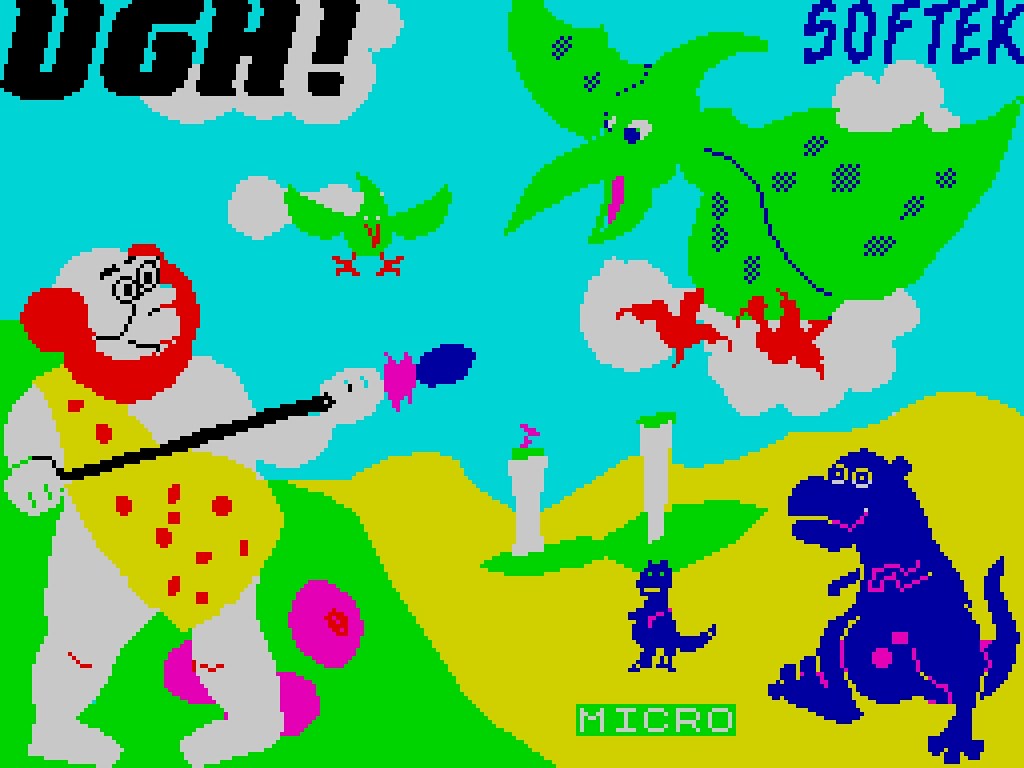In this vibrant video game scene, the word "UGG" is prominently displayed in the upper left corner in large, black, jagged letters, emphasizing a moment of frustration or surprise. The sky is a clear blue, dotted with gray clouds, and features a large, unique bird soaring through the air. This bird has striking big feathers, large ears, a pink beak, and distinctive webbed red feet. Flying in close formation behind it is a smaller, green bird, likely its baby, also sporting the same red webbed feet.

On the ground below, a caveman character with pale skin and round, eyeglass-like eyes stands ready for action. His appearance is slightly monkey-like, with a red beard and a primitive loincloth. He is armed with a sword-like weapon and surrounded by bright pink objects that resemble coconuts. Opposite him stands a menacing purple monster with blue highlights, accompanied by a smaller version of itself, adding a family dynamic to the scene. The overall image captures a whimsical and adventurous moment, filled with eccentric characters and vibrant details.